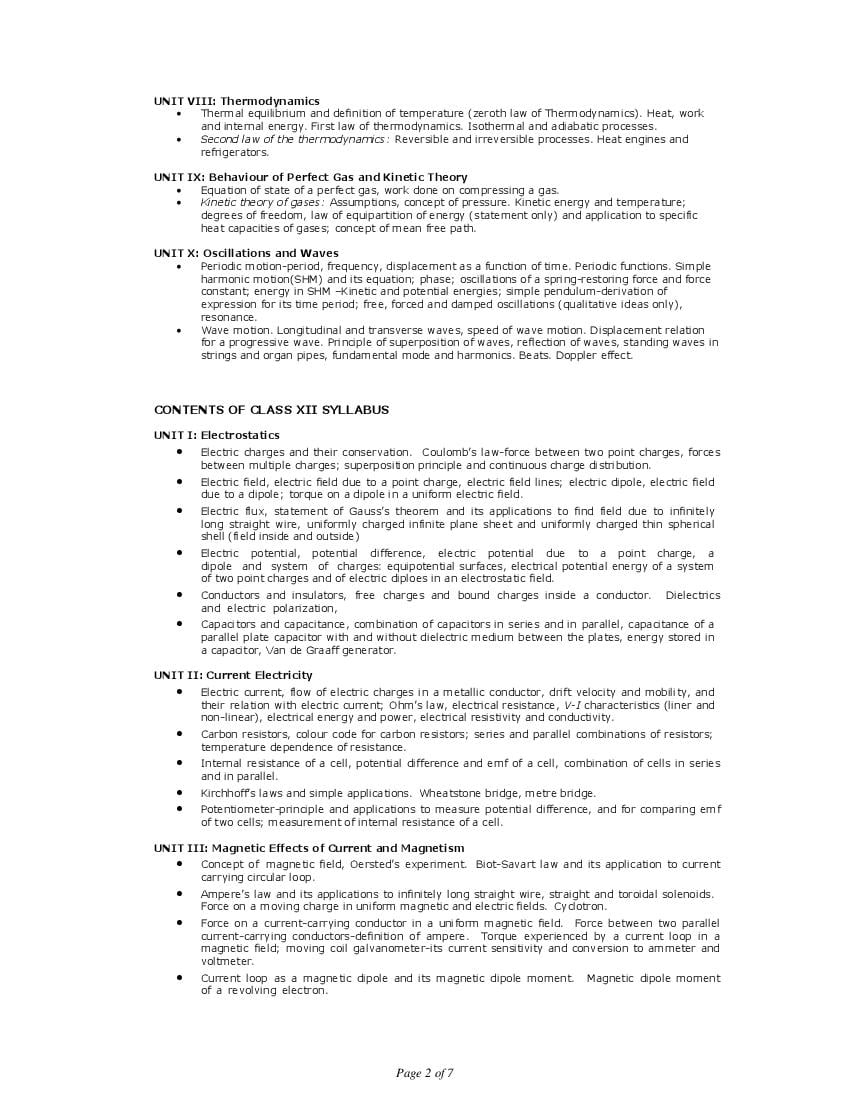**Title: Detailed Overview of Syllabus Content from Units 8 to 10 and Class 11-12**

**Image Description:**
The image presents a meticulously organized syllabus document printed in black ink on a completely white background. The content spans several key units and topics in physics, structured with bullet points and headings for clarity.

At the top, the document is titled "Unit 8: Thermodynamics." Each of the major topics within this unit is listed in bullet form, including:

- Thermal Equilibrium and Definition of Temperature
- 0th Law of Thermodynamics
- Heat, Work, and Internal Energy
- 1st Law of Thermodynamics
- Isothermal and Adiabatic Processes
- 2nd Law of Thermodynamics
- Reversible and Irreversible Processes
- Heat Engines and Refrigerators

Next, the document transitions to "Unit 9: Behavior of Perfect Gas and Kinetic Theory." Key points under this unit include:

1. Equation of State of a Perfect Gas
2. Work Done on Compressing a Gas
3. Kinetic Theory of Gases: Assumptions, Concept of Pressure, Kinetic Energy and Temperature
4. Degrees of Freedom
5. Law of Equipartition of Energy (Statement Only)
6. Application to Specific Heat Capacities of Gases
7. Concept of Mean Free Path

Following this, "Unit 10: Oscillations and Waves" is detailed. The key concepts under this unit are:

- Periodic Motion: Period, Frequency, Displacement as a Function of Time
- Periodic Functions
- Simple Harmonic Motion (SHM) and its Equation
- Phase
- Oscillations of a Spring: Restoring Force and Force Constant
- Energy in SHM: Kinetic and Potential Energies
- Simple Pendulum: Derivation of Expression for its Time Period
- Free, Forced, and Damped Oscillations (Qualitative Ideas Only)
- Resonance
- Wave Motion: Longitudinal and Transverse Waves
- Speed of Wave Motion
- Displacement Relation for a Progressive Wave
- Principle of Superposition of Waves
- Reflection of Waves
- Standing Waves in Strings and Organ Pipes: Fundamental Mode and Harmonics
- Beats and Doppler Effect

The next significant heading reads "Contents of Class 11, Class 12 Syllabus." This section begins with "Unit 1: Electrostatics," covering points like:

- Electric Charges and their Conservation
- Coulomb's Law: Force between Two-Point Charges, Forces between Multiple Charges, Superposition Principle, and Continuous Charge Distribution
- Electric Field: Due to a Point Charge, Field Lines, Dipole, Field Due to Dipole, Torque on a Dipole in a Uniform Field
- Electric Flux: Statement of Gauss's Theorem and its Applications
- Electric Potential: Potential Difference, Potential Due to a Point Charge and a Dipole, Equipotential Surfaces, Electrical Potential Energy
- Conductors and Insulators: Free and Bound Charges, Dielectrics, Electric Polarization
- Capacitors and Capacitance: Series and Parallel Combinations, Capacitance of Parallel Plate Capacitors, Energy Stored, Van de Graaff Generator

"Unit 2: Current Electricity" follows, including:

- Electric Current: Flow of Charges, Drift Velocity, Mobility, and Relation with Current
- Ohm's Law: Electrical Resistance, V-I Characteristics (Linear and Non-Linear), Electrical Energy and Power
- Electrical Resistivity and Conductivity: Carbon Resistors, Color Code, Series and Parallel Combinations, Temperature Dependence
- Internal Resistance of a Cell: Potential Difference and EMF, Series and Parallel Combinations, Kirchhoff's Laws, Wheatstone Bridge, Meter Bridge, Potentiometer, Measuring Internal Resistance

Lastly, "Unit 3: Magnetic Effects of Current and Magnetism" entails:

- Concept of Magnetic Field: Ørsted's Experiment, Biot-Savart Law, Ampère's Law, Applications
- Force on Moving Charges: Uniform Magnetic and Electric Fields, Force between Current-Carrying Conductors, Definition of Ampère, Current Loop in a Magnetic Field, Moving Coil Gavinometer
- Magnetic Dipole Moment: Current Loop, Revolving Electron

At the bottom center of the image, the document indicates "Page 2 of 7."

This detailed syllabus describes fundamental and advanced concepts essential for physics students, offering a thorough and organized guide across multiple units.